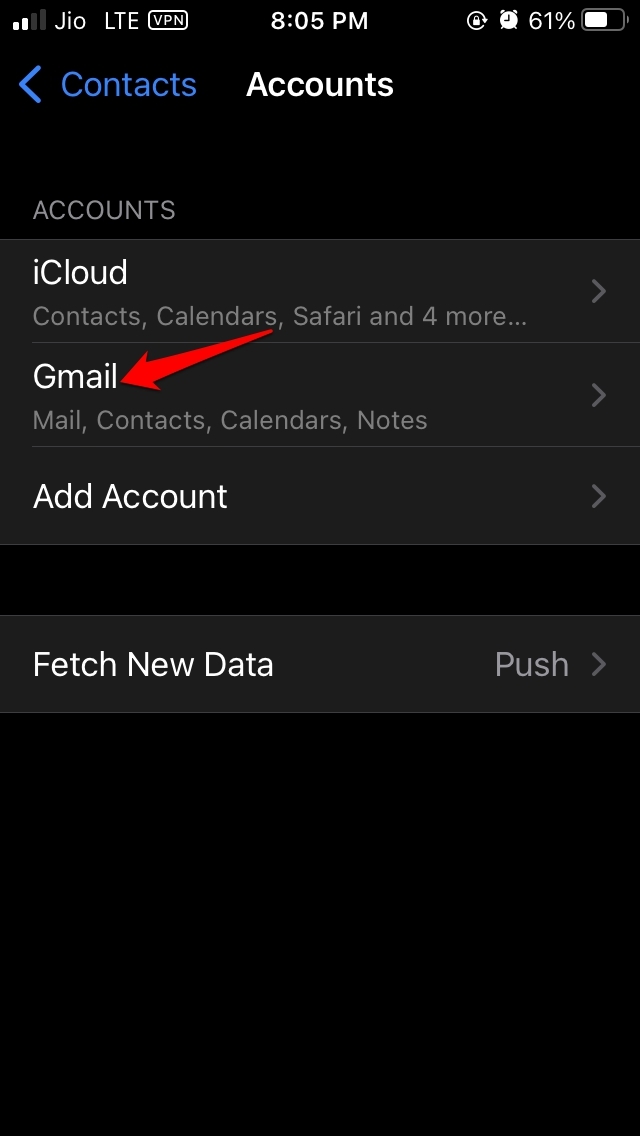This is a detailed screenshot of a cell phone interface with a black background. The status bar at the top shows network details: two out of four signal bars are white while the other two are dark. The network provider is labeled as "JIO LTE," and a VPN icon is displayed in a square. The current time reads 8:05 PM. To the right of the time, there are icons for a secured lock, an alarm, a battery level indicator showing 61% charge, and the numeric percentage itself.

Below the status bar, the interface has a blue heading labeled "Contacts" with an arrow pointing to the left. In the center, the bold white text reads "Accounts." Beneath this main heading, a lighter gray bar with the text "Accounts" is followed by several account options.

The first option is "iCloud," displayed in white. Under "iCloud," the options listed are Contacts, Calendars, Safari, and an indicator of four more items. The next account option is "Gmail," also in white, followed by Mail, Contacts, Calendars, and Notes. A prominent red arrow points to the Gmail option for emphasis.

After these account options, there is an "Add Account" selection. Below this, a black bar delineates the end of this section. Further down, white text reads "Fetch New Data," with the word "Push" and a right-pointing arrow displayed to its right. Each account option, including iCloud, Gmail, and Add Account, has an arrow on the right-hand side indicating a navigable link or further options.